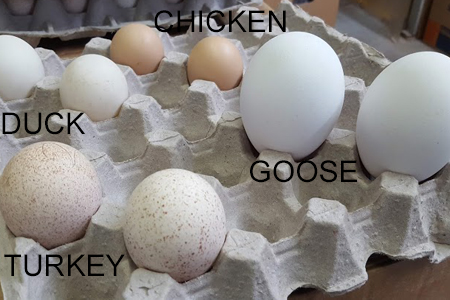The image depicts an open light gray egg carton with compartments for holding eggs. Inside the carton, eight eggs are neatly arranged in pairs, each pair labeled with black text denoting their type. Starting from the bottom left corner, there are two beige, polka-dotted turkey eggs labeled "turkey." Directly above them to the left middle are two smaller, regular white eggs labeled "duck." Further up to the top middle-left, there are two light brown chicken eggs with "chicken" written above them. Finally, on the top right corner are two large white eggs labeled "goose." The carton is slightly tilted with the left side angled slightly towards the camera, offering a clear view of the labeled arrangement of the eggs.